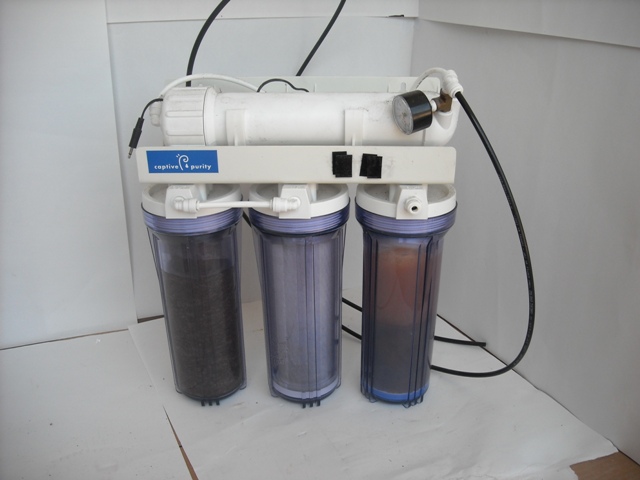This image captures a close-up view of a water filtration system designed for under-sink installation. The system features three main plastic canisters, each filled with different fluids visible through their clear casings: the leftmost canister has a darker fluid, the middle one appears to be either silver or empty, and the rightmost contains a lighter, orange-hued fluid. Above these three canisters, a fourth horizontal white tube stretches across, indicative of a fourth filtration stage. The digital image is set against a backdrop of white paper, likely to protect a brown wooden surface visible at the edges, suggesting potential wetness of the area. Additionally, more white paper is taped to the wall behind the unit, emphasizing the clean, clinical setting. Cords and cables in the background hint at connections for power or auxiliary functions, enhancing the detailed setup of this water filtration apparatus.